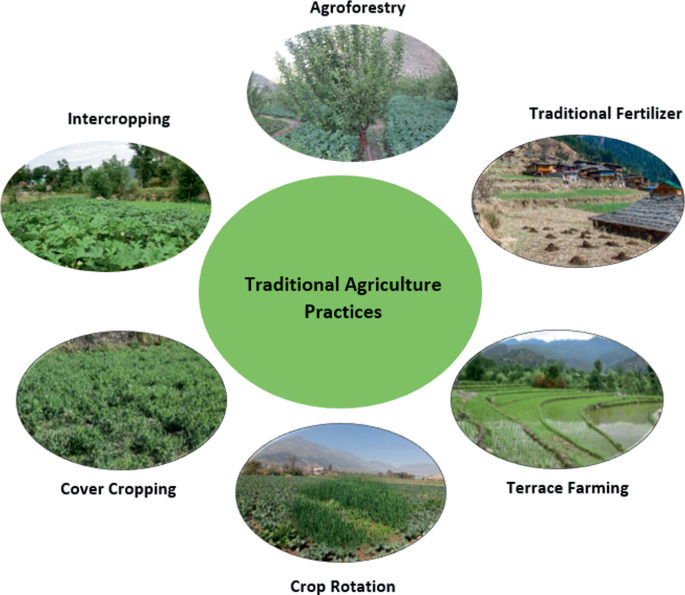The image depicts a central green circle with black text reading "Traditional Agricultural Practices." This central circle is surrounded by six smaller circles, each representing a specific practice and arranged to form a hexagonal pattern. Starting from the top and moving clockwise, the circles are labeled as follows:

1. Agroforestry: Shows a tree with rows of green crops behind it.
2. Traditional Fertilizer: Depicts cultivated land with green steps and brown mounds.
3. Terrace Farming: Features a green field with ridges and water channels.
4. Crop Rotation: Displays a green field filled with crops.
5. Cover Cropping: Shows a dense cover of overgrown plants.
6. Intercropping: Illustrates a field with diverse crops.

Each smaller circle includes a corresponding color photograph that visually represents the described agricultural practice, emphasizing the lush green vegetation characteristic of these traditional methods.